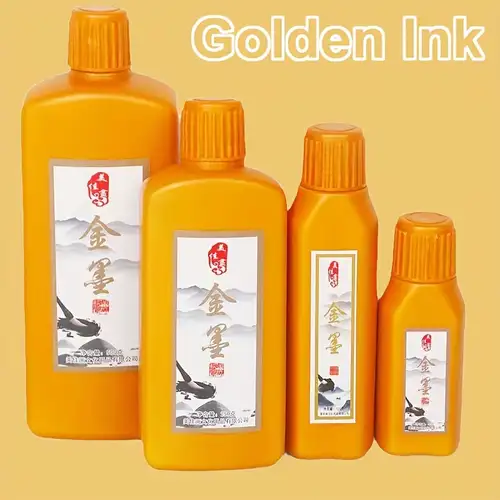The image is an advertisement featuring four golden bottles, arranged in descending order of height from left to right. The backdrop is a light orange or golden hue, complementing the more vibrant orange of the bottles. Each bottle has a twist top in a darker shade of orange. The largest bottle stands at the left, graduating down to a travel-size bottle on the right. The bottles are categorized by shape: the two larger bottles have rounded shoulders, while the two smaller ones have a different top configuration.

All four bottles are nearly identical save for their size, with white labels trimmed in silver. These labels feature gold Japanese writing framed by two red insignias. Additionally, there's a basic design on the labels that includes black mountain tops and possibly a brush stroke extending from the left. The only legible text is "GOLDEN INK" written in white outline on the top right of the advertisement, suggesting the bottles may either be cosmetic products or related to painting, as hinted by the imagery of the paintbrush on the label.